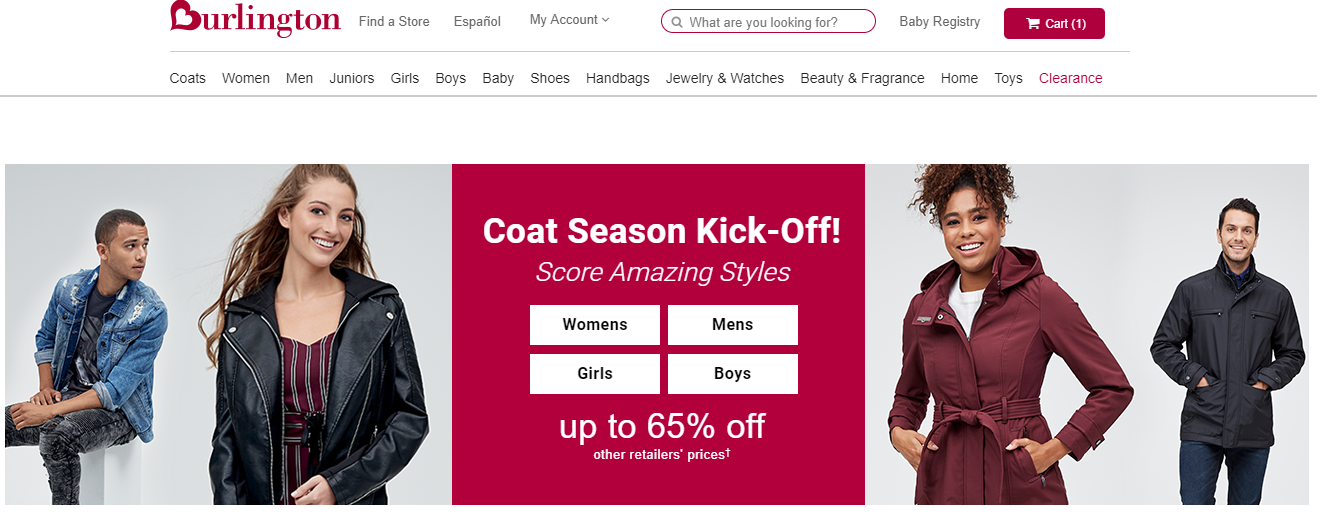This is a detailed and cleaned-up caption based on the description provided:

---

The screenshot captures a section of the Burlington website, specifically the header and part of the homepage. The background is white and the layout is notably wider than tall. 

At the top left, the Burlington logo features a heart on its side resembling the letter "B" in burgundy font, with "Burlington" written to its right. Adjacent to the logo, in smaller black text, are the options: "Find a Store," "Español," and "My Account" with a dropdown menu. Completing the top bar is a search bar with a magnifying glass icon, a baby registry link, and a red shopping cart icon showing one item inside.

Below this navigational bar are multiple categories in a horizontal menu, including "Coats," "Women," "Men," among others, totaling around ten options. The last category, "Clearance," is highlighted in red while the others remain black, indicating it has been selected.

The main body below the category tabs features two side-by-side promotional images—each containing a stylishly dressed man and woman. Separating these pictures is a red box with the text "Coat Season Kickoff" and "Core Amazing Styles." It highlights a discount of "up to 65% off" and includes four navigation buttons arranged in a square for "Women," "Men," "Girls," and "Boys."

---